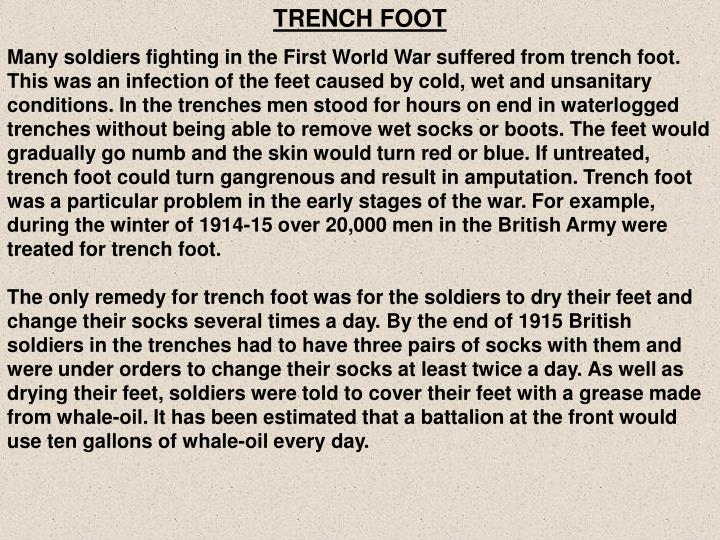The image appears to be a scanned slide or PowerPoint presentation with a beige background and bold, black Arial font text. At the top, the title "TRENCH FOOT" is prominently displayed in all capital letters, underlined for emphasis. Below the title, two detailed paragraphs describe Trench Foot, an infection many soldiers suffered from during the First World War due to the cold, wet, and unsanitary conditions in the trenches. Soldiers often stood for hours in waterlogged trenches, unable to remove their wet socks or boots, which caused their feet to go numb, turn red or blue, and potentially become gangrenous, sometimes necessitating amputation. The text highlights that during the winter of 1914-15, over 20,000 British soldiers were treated for Trench Foot. The only remedy was for soldiers to dry their feet and change their socks several times a day. By the end of 1915, British soldiers were required to carry three pairs of socks and were instructed to change them at least twice daily, often applying whale oil to their feet, with battalions reportedly using 10 gallons of whale oil per day. The detailed text, covering the entire image area, suggests its use in an educational setting.